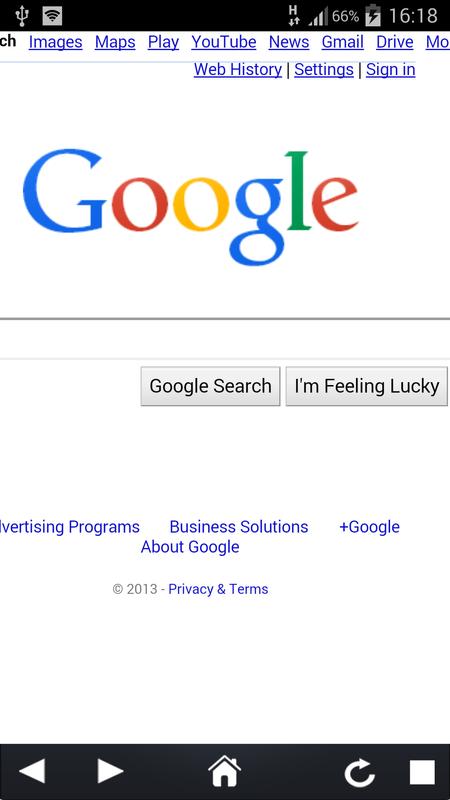This image depicts a smartphone screen with an active USB connection, indicated by the corresponding icon. The phone's Wi-Fi is enabled, and both uploads and downloads are in progress, as shown by the status indicators. The battery level is displayed at 66%, and the time is 16:18. 

The top of the screen features a black bar with various Google service links: Images, Maps, Play, YouTube, News, Gmail, Drive, Web History, Settings, and Sign-in, all in clickable blue text. 

Beneath this bar, the Google logo stands out in its classic branding colors: a blue capital 'G' followed by a red 'o', yellow 'o', blue 'g', green 'l', and red 'e'. Under the logo, there is a partially visible search bar with the buttons "Google Search" and "I'm Feeling Lucky" positioned below it.

Further down, the screen displays several text links in small font: Advertising Programs, Business Solutions, Google+, and About Google, followed by "2013 Privacy and Terms." 

At the very bottom of the screen, the phone's navigation bar includes icons for the home screen, refresh, and forward and back arrows, providing additional navigation options.